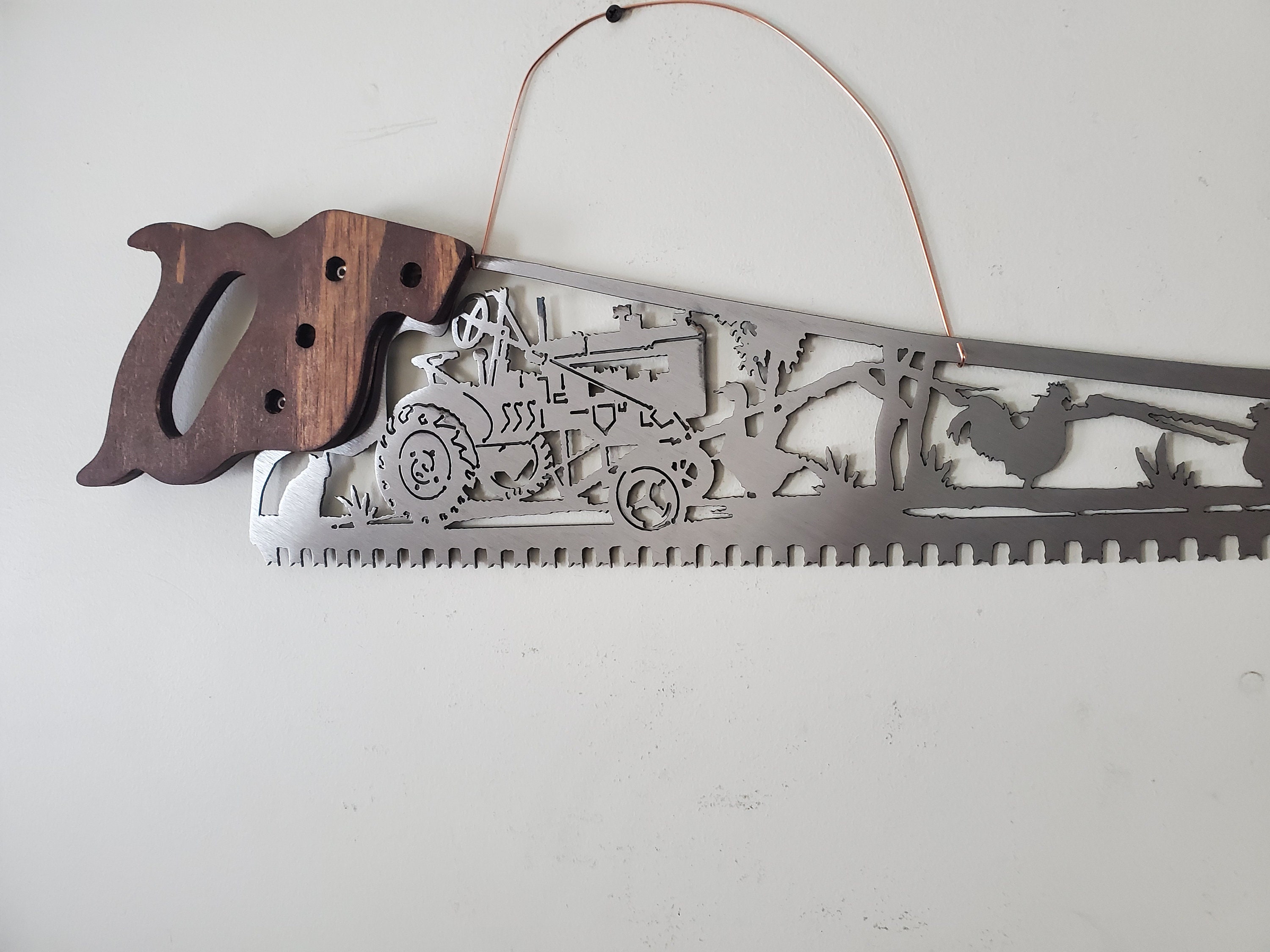In this color photograph, a uniquely designed wood saw hangs on a white-painted wall, suspended by a metal wire from a nail. The saw, which boasts a traditional wooden handle, features intricate carvings along its blade. These carvings depict a detailed farm scene, complete with a tractor, ducks, chickens, and a tree set against a grassy backdrop. The saw has large teeth, typical of those used to cut large pieces of wood, but its ornate design transforms it into a piece of art rather than a functional tool.